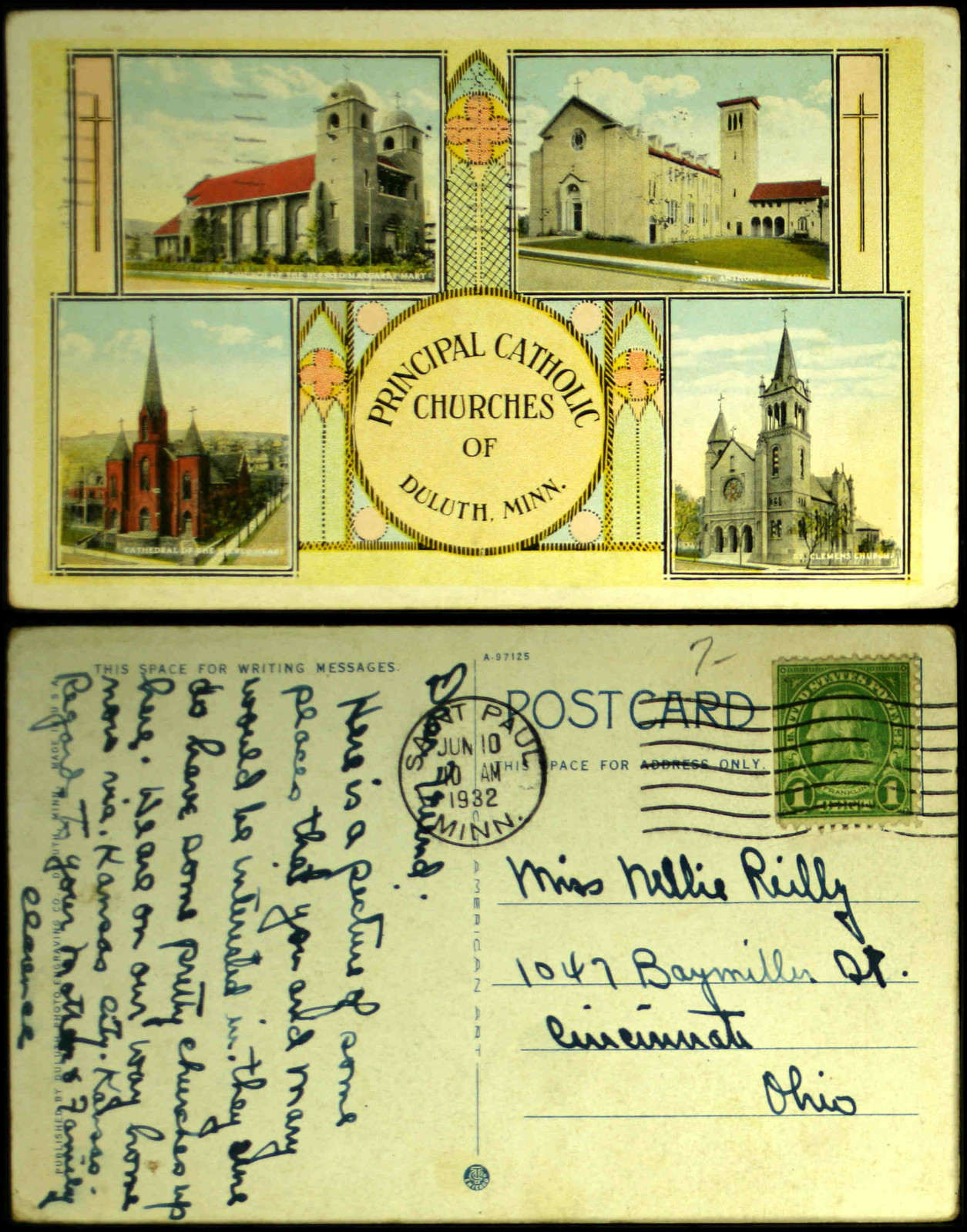The image displays both the front and back of a historical postcard within a single 8x10 piece of paper. The top half showcases the front of the postcard, which is a horizontal rectangle featuring four old photographs of churches. These images are collectively labeled "Principal Catholic Churches of Duluth, Minnesota." The top two photographs do not have arches, while the bottom two boast gothic architecture with pointy rooftops. The bottom half of the image reveals the back of the postcard, addressed to "Miss Nellie Riley, 1047 Baymiller Street, Cincinnati, Ohio." The postcard has a green one-cent stamp in the upper right corner, postmarked from St. Paul, Minnesota, on June 10, 1932, at 10 a.m. Written in dark blue or black ink, the message reads: "Dear Friend, here is a picture of some places that you and Mary would be interested in. They sure do have some pretty churches up here. We are on our way home now via Kansas City, Kansas. Regards to your mother and family, Clarence."